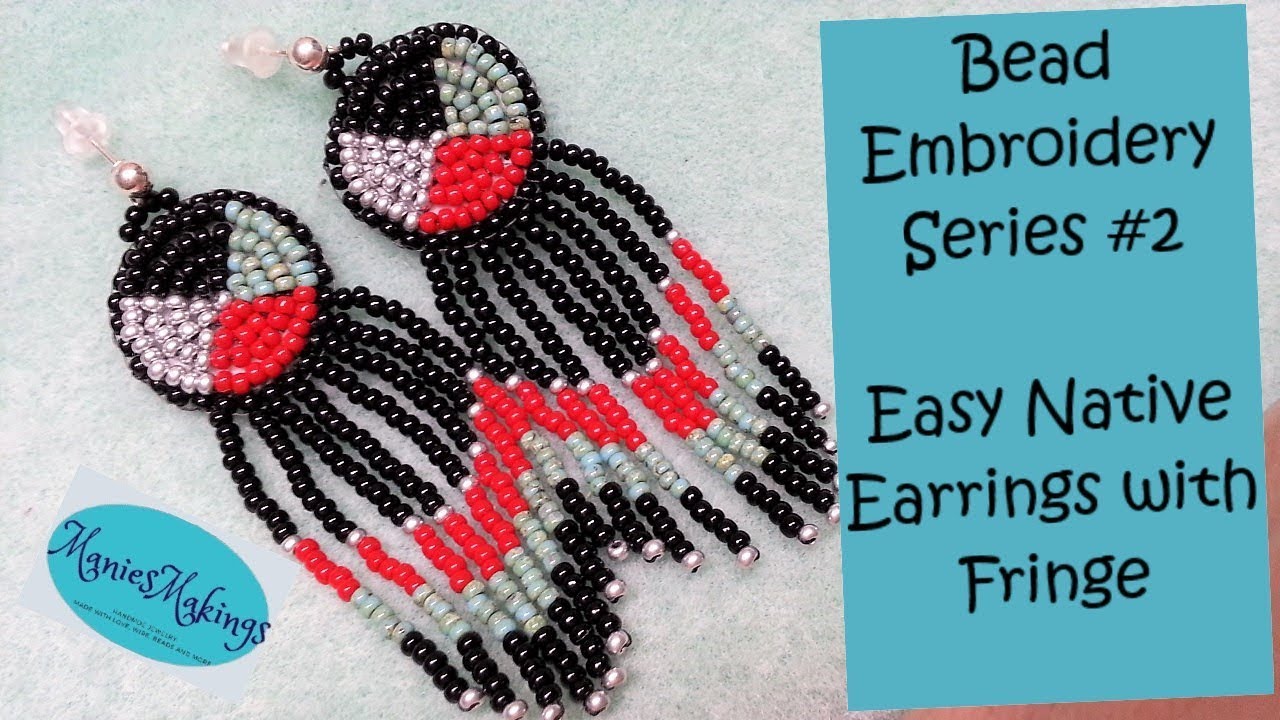This horizontal photograph showcases a pair of meticulously handcrafted Native American-inspired beaded earrings resting on a light-colored textured surface, possibly white or pale mint green. Each earring features a circular top segment adorned with wedge-shaped sections of red, black, mint green, and silver beads. Below the circular design, eight intricate beaded fringes extend downward. The fringes begin with a strip of black beads, followed by a silver bead, a stretch of red beads, mint green beads, another stretch of black beads, and finally a single silver bead at the bottom. 

These earrings are designed for pierced ears, equipped with hooks at the very top. The image contains a blue oval sticker in the lower left corner reading "Maney's Makings," and a blue rectangular label on the right side with the text "Bead Embroidery Series Number Two, Easy Native Earrings with Fringe."